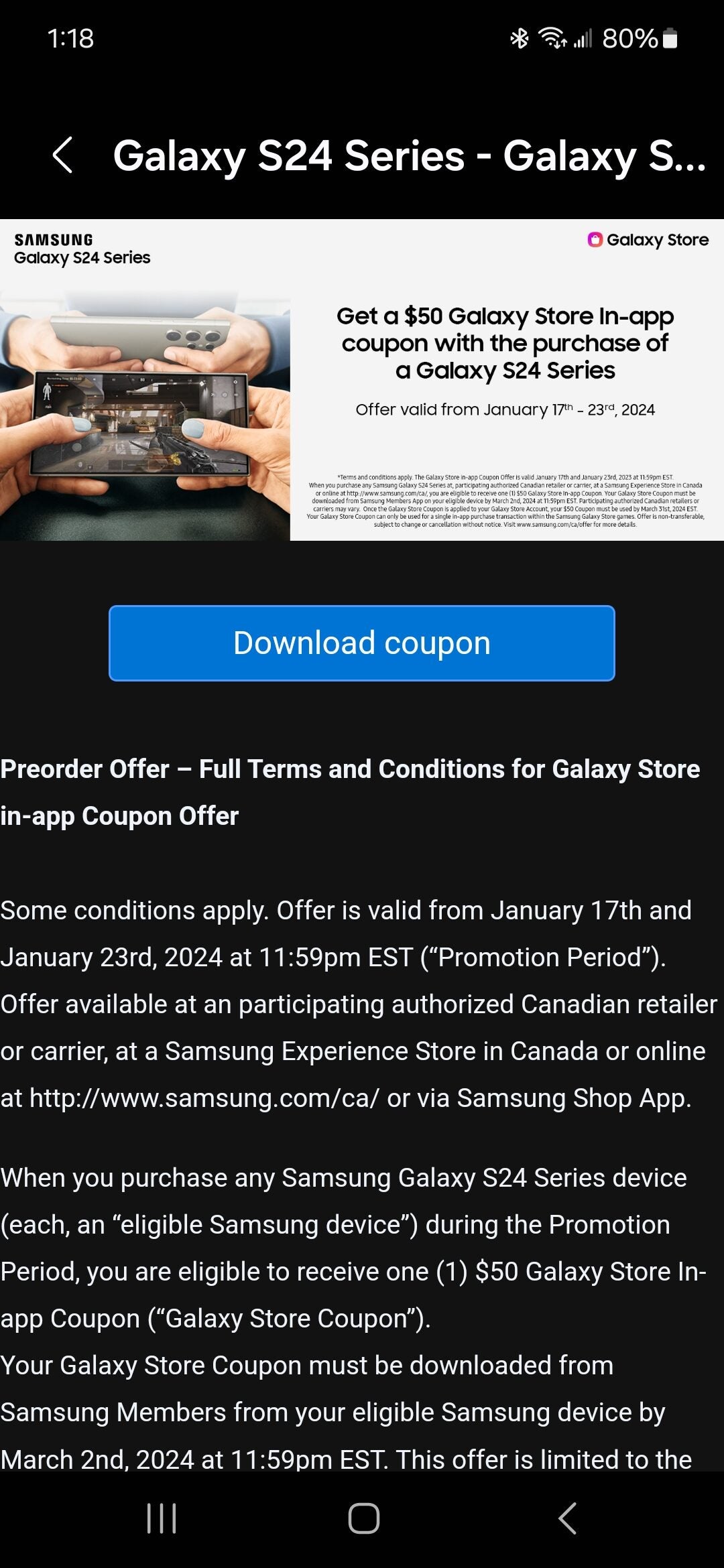This screenshot, captured on a mobile device, showcases a promotional page predominantly designed in black with white text at the top reading "Galaxy S24 series." Below this header is an advertisement featuring the Galaxy S24 device held in someone's hands. The ad prominently states, "Get a $50 Galaxy Store in-app coupon with the purchase of a Galaxy S24 series." Beneath this advertisement, there is a prominent blue button labeled "Download Coupon." Further down, detailed terms and conditions for the coupon offer are visible in smaller text. The sleek design and concise information make the promotion visually appealing and easy to understand.